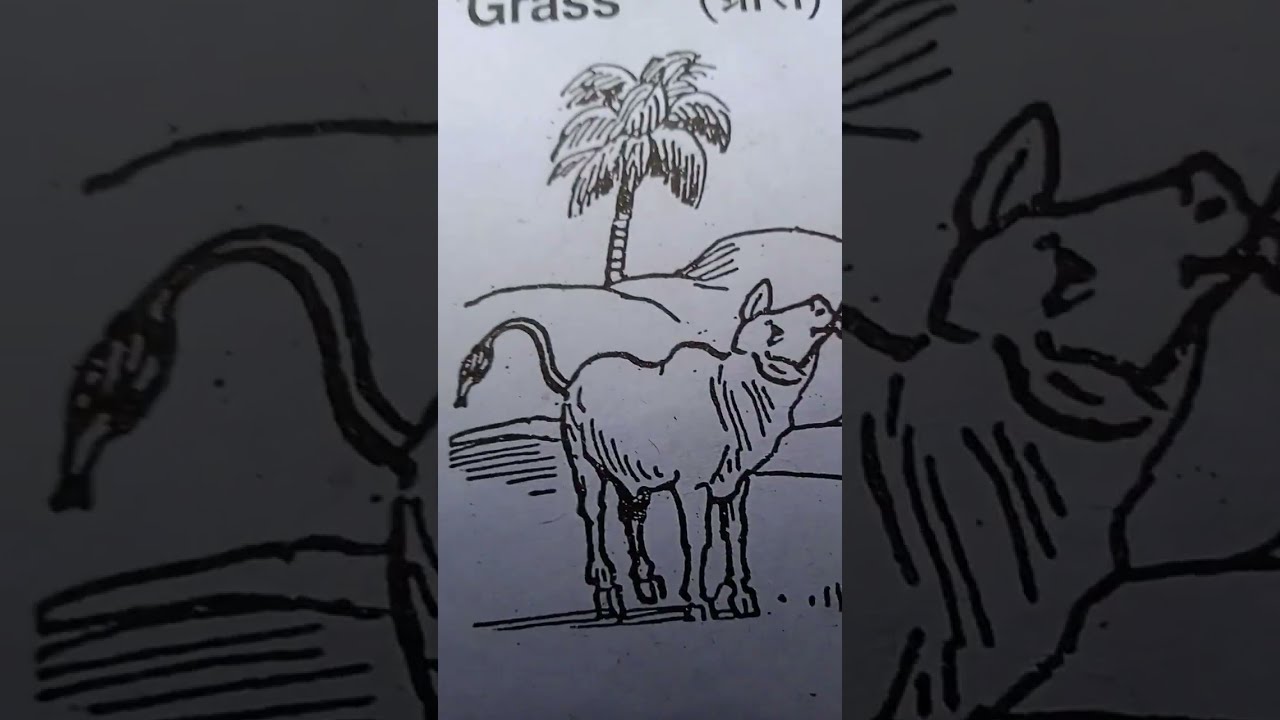The black-and-white image appears to be a hand-drawn illustration from a children's book, characterized by its simple, pencil-like or marker-drawn lines. The central figure is likely a cow or a lamb, with its head tilted upward, gazing towards the sky at an approximate 1 o'clock position. Its tongue is sticking out, adding a sense of action or engagement with its surroundings. The animal's ears and eyes are clearly visible, and its tail is lifted in the air. The background features a single palm tree with detailed lines on its trunk, and some rolling hills. The word "grass" is prominently placed in the upper left, although partially cut off, and there's an indecipherable word in parentheses in the upper right. The composition of the image seems to be divided into three sections, with the central section being the main focus and the adjacent sections darkened and zoomed in to highlight details. The illustration, devoid of any complex textures, likely serves an educational purpose, aiming to help children recognize and learn words and objects.